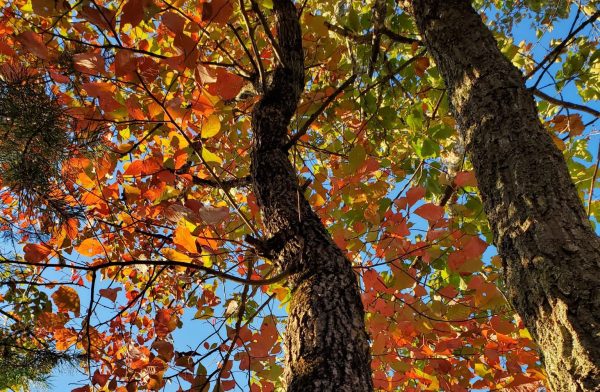This vibrant photo captures a towering tree, possibly two, taken from a ground-up perspective. It feels as though the viewer is lying on the ground, gazing skyward through the canopy. The tree trunks, appearing gray and bumpy with peeling bark, support a cascade of thin, spindly branches adorned with a mosaic of leaves. These leaves display a stunning array of colors—predominantly orange, yellow, and green, with a scattering of golden and red hues—suggestive of a crisp fall day. The clear blue sky, visible through the leaves, provides a perfect backdrop, with no clouds in sight. Sunlight filters through the leaves and branches, casting a glistening effect that enhances the natural beauty of this serene, daytime scene.